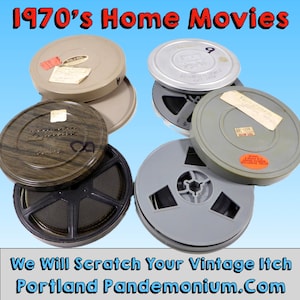This advertisement, presented as a small square image, vividly evokes nostalgia with its 1970s theme. Set against a light blue sky background, the centerpiece consists of old-style reel-to-reel film canisters, akin to those used with vintage projectors. At the top, bold red text reads "1970s Home Movies," capturing the essence of the era. The canisters, eight in total, are spread across the image in two vertical columns and varying positions, showcasing a variety of colors and conditions from gray, black, and silver to more unique hues like light brown, red, and blue. Some canisters are open, revealing the black film reels inside, and several display paper stickers or handwritten labels, including one with the number '9'. Towards the bottom, a gray rectangle contains blue text that promises, "We will scratch your vintage itch, Portland," followed by the website address "portlandpandemonium.com." This visually engaging advertisement invites viewers to reminisce and potentially revisit or restore cherished home movie memories.